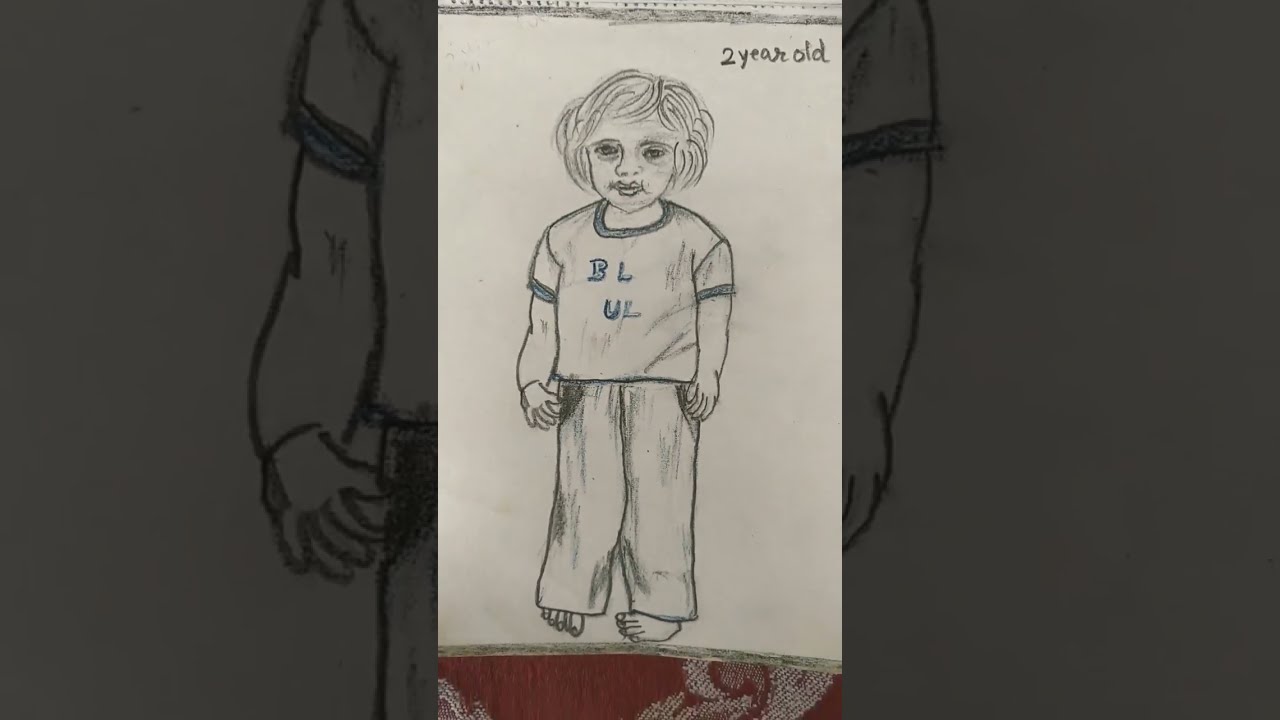The image is a detailed pencil sketch on a piece of white paper, still attached to a sketch pad, as evidenced by the visible spiral holes at the top. It depicts a young child with short, slightly flyaway hair styled in a bob. The child has a babyish, pudgy face and is wearing a short-sleeved t-shirt that reads "B.L.U.L." along with baggy pants. The child is barefoot, with one foot turned inward and the toes of the other foot just visible. The sketch has a smudgy appearance, likely from the pencil markings being smeared. At the top right corner of the paper, it says "2 year old." Below the image, there is an area with a red and white design. Surrounding the main drawing, the same image is enlarged, grayed out, and used to create a border. The entire drawing is in black and white, without any added color.